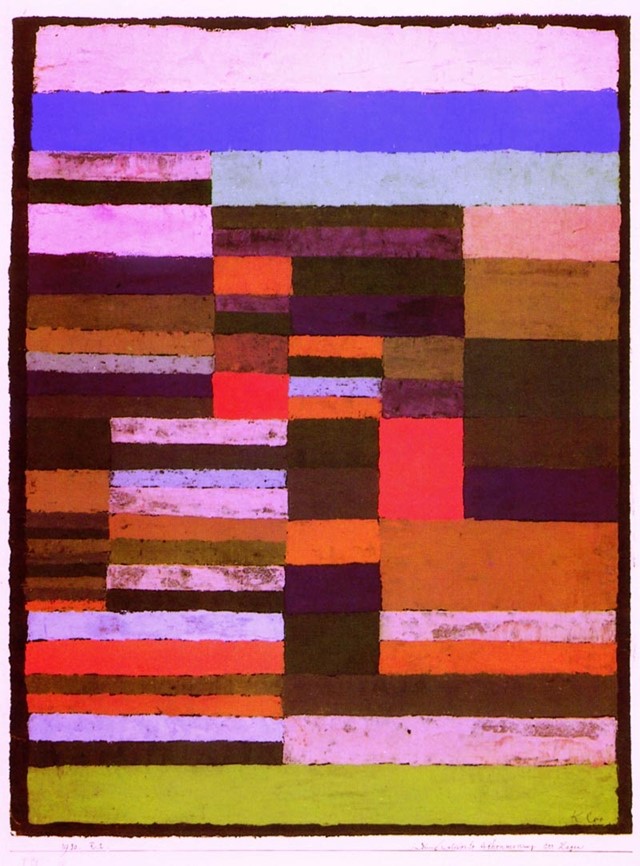This image features a vertically oriented rectangle that initially evokes the appearance of a large rug or a piece of modern art. The composition is meticulously color-blocked, showcasing a diverse array of colored stripes and rectangles in various sizes and patterns. The dominant hues consist of light pink, blue, and purple, with accents of darker pink, orange, green, and multiple shades of brown. 

The first row at the top is narrow, encompassing a pink block, followed by a similarly sized purple block. Below that, a larger section includes stacked pink and brown rectangles covering about a quarter of the total height, alongside a more extensive gray area. As you progress downward, alternating color patterns become evident, featuring combinations of pink, brown, red, dark brown, burgundy, and orange in varying arrangements. 

One noteworthy element is a distinct lime green stripe at the bottom, adding a vivid contrast absent from the rest of the artwork. The structured layout of lines and color divisions contributes to a visually dynamic piece. Although it might initially resemble a textile, the detailed brushwork and color application suggest it is more likely a painting, potentially inspired by textile patterns. The signature in the bottom right corner appears to read something like "K," although the exact artist's name remains unclear.